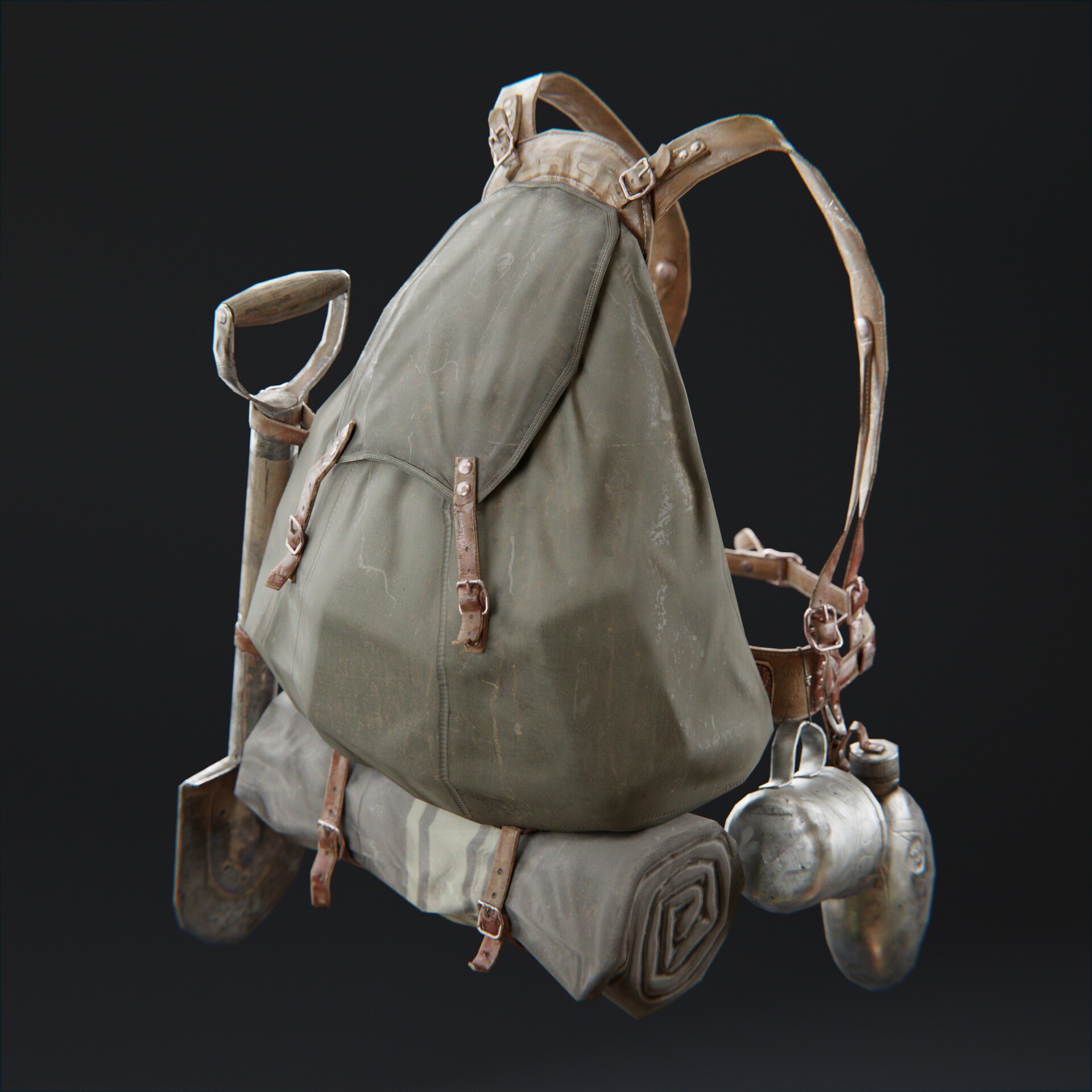This image showcases an antique camping or military kit, likely from the 1930s or 1940s. The centerpiece is a large, triangular, olive drab canvas backpack with brown leather shoulder straps attached via belt buckles. Below the backpack, a rolled-up blanket is securely fastened using leather belt straps. The setup is further detailed by various attached items: on the right side, a steel cup and canteen hang from clips, and on the left side, a small shovel is fastened with a leather strap. The overall composition, with its muted, rustic colors and functional design, underscores the vintage and utilitarian nature of this historic gear.